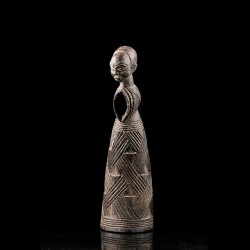In this image, we see an ancient African idol doll positioned against a stark black background, perhaps displayed on a table or in a museum showcase. This statue is crafted from a metal resembling bronze or copper, giving it a brownish hue. The figure, likely depicting a woman, features a prominently larger head, adorned with short, cropped hair. The body is shaped almost like a cone, resembling a long, sleeveless robe with intricate line details etched into the dress. Notably, the doll is missing its arms, which appear to be broken. The head is slightly turned over the shoulder, facing left, and there is a reflective surface visible beneath the statue, enhancing its display. The doll has a hole in the chest, adding to its ancient and enigmatic appearance.